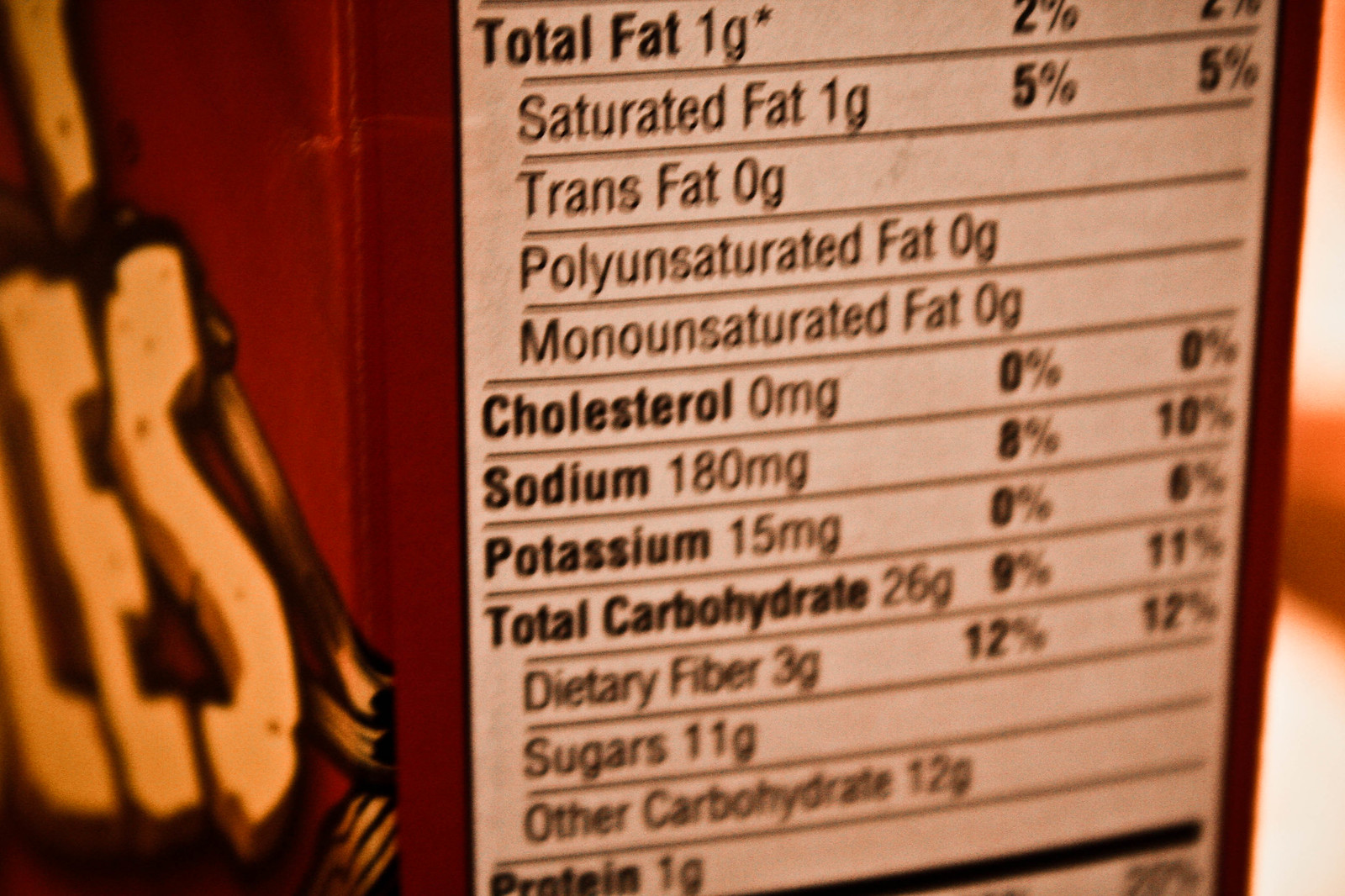The image showcases a nutrition label on the side of a box, likely that of Fruity Pebbles cereal, identifiable by partial letters "E" and "S" against a vivid red background. The letters appear in a distinctive, somewhat sloppy gold script. The label provides detailed nutrition information: total fat is 1 gram, with specifics on saturated fat (1 gram), trans fat (0 grams), polyunsaturated fat (0 grams), and monounsaturated fat (0 grams). Also listed are cholesterol (0 milligrams, 0%), sodium (180 milligrams), potassium (15 milligrams), and in bold text, total carbohydrate at 26 grams, with dietary fiber at 3 grams, sugars 11 grams, and other carbohydrates 12 grams. The label concludes with protein content at 1 gram, displayed in black text.